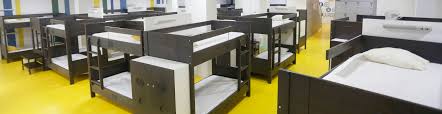This is a detailed photograph taken in what appears to be a furniture store or warehouse, showcasing rows of bunk bed displays. The room features a bright yellow floor and white walls accented with blue and yellow stripes. Each bunk bed has a uniform dark frame, described variously as black, dark gray, or dark brown, with safety railings on the top bunks. The beds are all twin-sized and feature attached ladders, either on the right or left side. Each bunk bed includes a white mattress, pillows with white pillowcases, and some form of storage unit or cabinetry built into the side. The layout includes multiple aisles of these bunk beds, all arranged in neat rows, echoing the style and model consistently. The photo gives an impression of a spacious showroom, similar to places like Ikea, filled with identical rectangular loft-style bunk beds evidently aimed at children or small individuals.